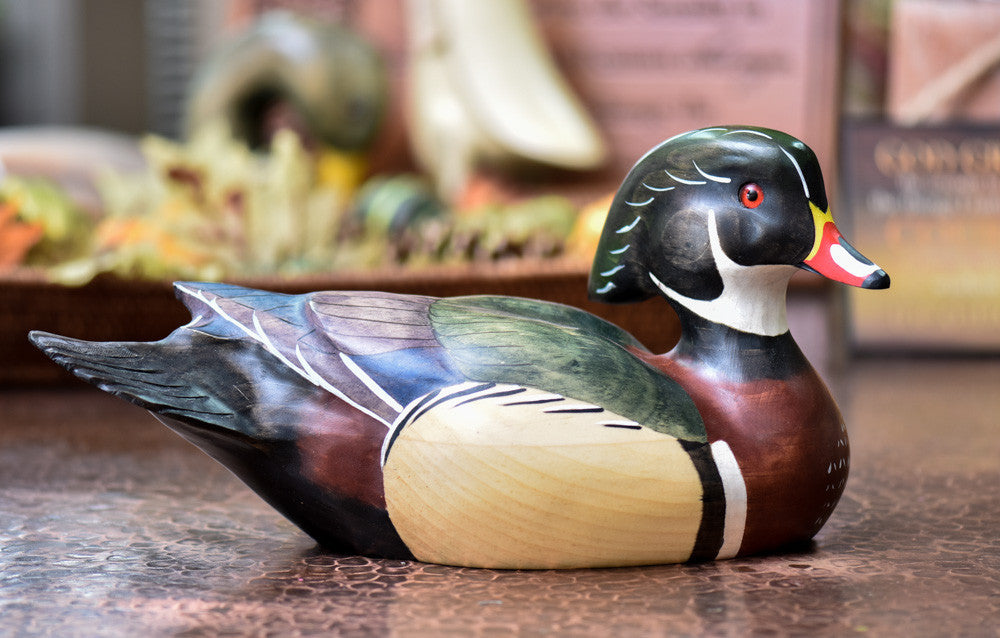This is a detailed photo of a meticulously carved wooden mallard duck decoy, perched on a brown countertop. The background is artfully blurred, drawing full attention to the exquisitely crafted duck, which appears as if it's gliding on water. The duck is facing right, with its tail extending left and resting flatly on the surface without any visible legs. 

The decoy features a complex palette: its beak vividly combines red, white, black, and yellow hues. The head is primarily black, adorned with iridescent green feathers towards the back. Its eyes have a striking red iris with a dark black pupil. Below its head, the duck's chin area is painted white, complemented by two white stripes on the neck, with a thin black line separating the head from the body. 

The body of the duck displays an artful mixture of colors—brown feathers on the breast, ivory and light brown on the flanks, and a combination of green, blue, and pink feathers adorning the wings. The tail is a dark charcoal black, extending straight out. 

The background suggests a cozy indoor setting with blurred household items, perhaps indicating the duck serves as a decorative element in someone's home. The precise carving and detailed paintwork highlight the craftsmanship of this beautiful wooden decoy replica, traditionally used for duck hunting.